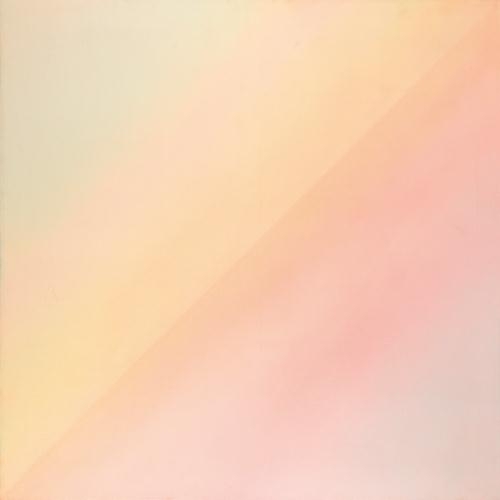"Afternoon in September" by Jeff Verheyen, created circa 1971, is a square-format, post-painterly abstraction painting characterized by its soothing gradient of blended colors and a diagonal crease running across the image. The composition transitions from a dark brownish-green in the top left corner, through shades of light peach, golden yellow, and rose, to predominantly pink tones with hints of light orange, blue, and green tints. The hues gently blend into one another, creating a cotton-like texture. The bottom right corner settles into a very light pink with a touch of whiteness, evoking a serene and reflective atmosphere.